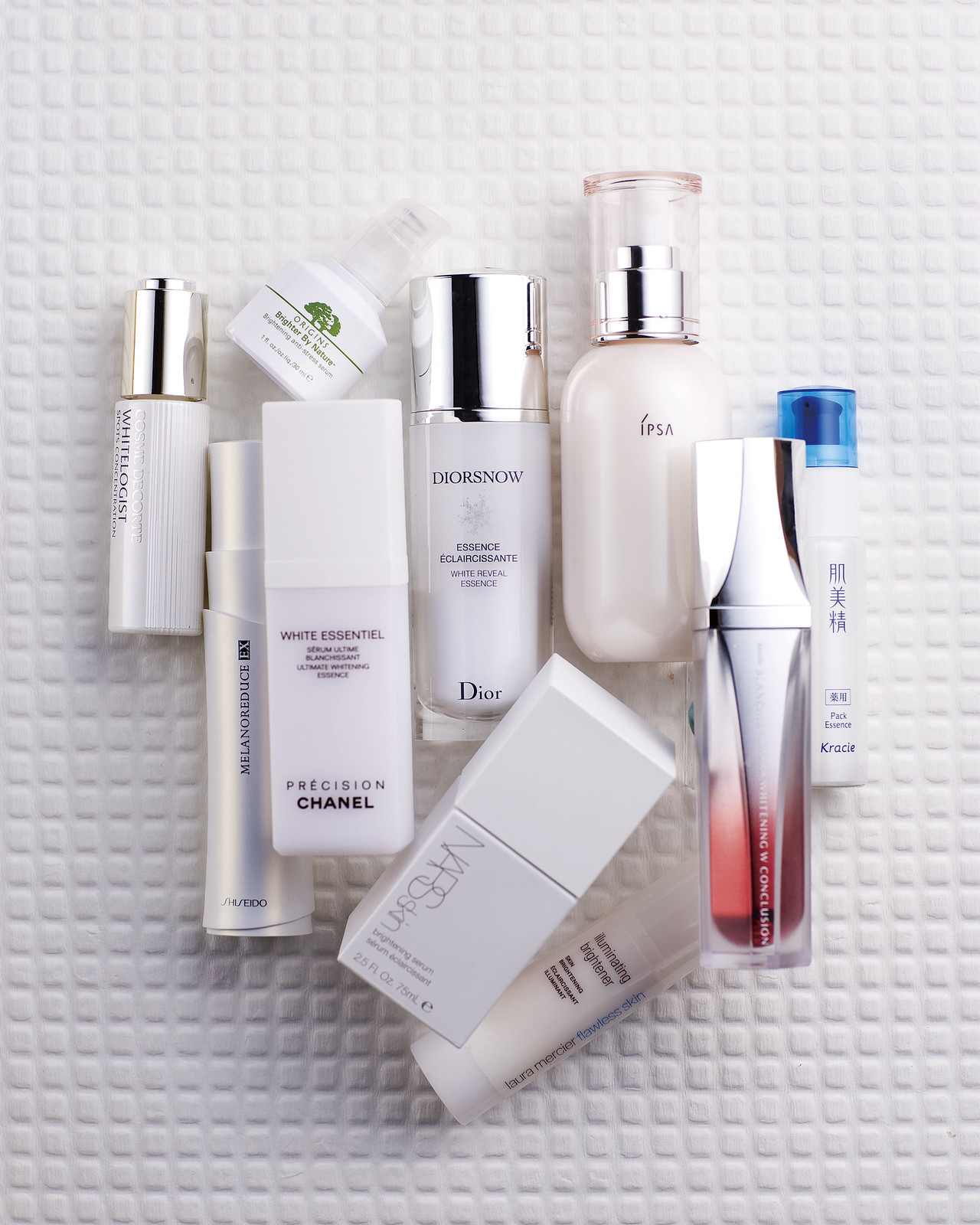The image appears to be an advertisement for various high-end cosmetic products artfully arranged on a white, textured, quadricular surface. The background grid of square tiles adds a tactile element to the display, drawing attention to the sleek and luxurious packaging of the products. The majority of the cosmetics are adorned in sophisticated white and silver tones, providing a modern and clean aesthetic. Notably, a mascara positioned on the right introduces a pop of color with a red accent on its lower portion. Additionally, a product with a distinctive blue lid breaks the monochromatic theme subtly. The image showcases an array of prestigious brands including Dior, Nars, Chanel, Shiseido, and IPSA, exemplifying a curated collection of premium beauty essentials. The bright and predominantly white composition emphasizes a sense of purity and elegance, characteristic of a high-quality advertisement.